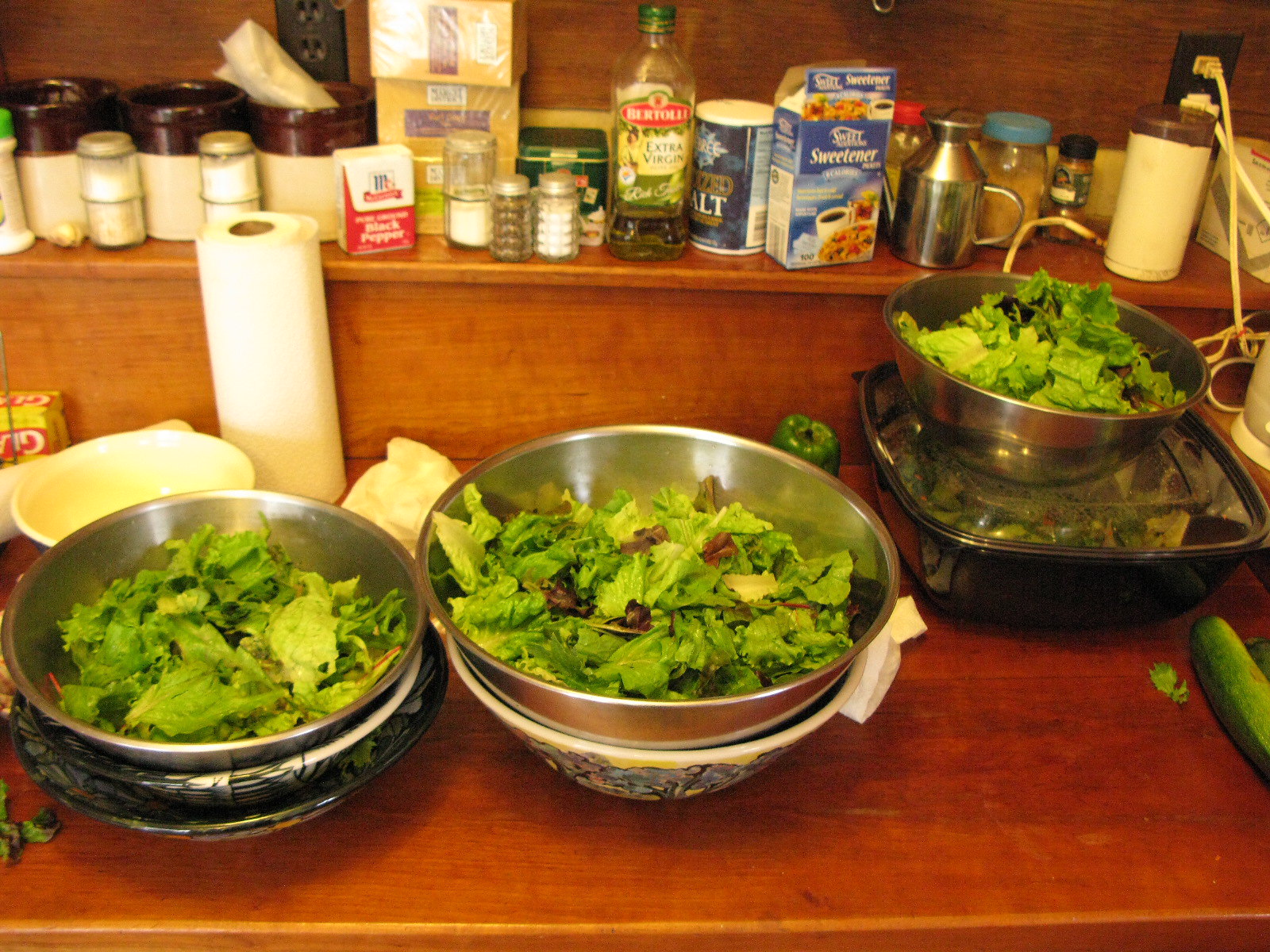In this detailed kitchen scene, various food prep items are arrayed on stepped, light reddish-brown shelves. The scene is centered around salad preparation, with multiple containers featuring torn romaine lettuce. In the foreground, there are two colanders each filled with torn lettuce, presumably for rinsing. Next to these is a large plastic basin that holds a metal bowl, also containing lettuce. In addition, there's a covered bowl with green contents, potentially broccoli or another green vegetable. Spreading across the counter, there is a whole cucumber, a green pepper, and a roll of paper towels standing upright. 

Higher up, the shelves display a mix of kitchen essentials including a bottle of Bertolli extra virgin olive oil, a cylindrical salt container, black pepper, a coffee sweetener box, and what appears to be tea bags. Also present are three brown ceramic jars, which seem to be empty, sitting neatly in front of an electrical socket. The setup extends to another electrical socket with two plugged-in cables, likely connected to a kettle just outside the frame. This well-organized, bustling kitchen clearly shows someone in the midst of preparing a fresh and vibrant salad amidst a variety of other kitchen staples.